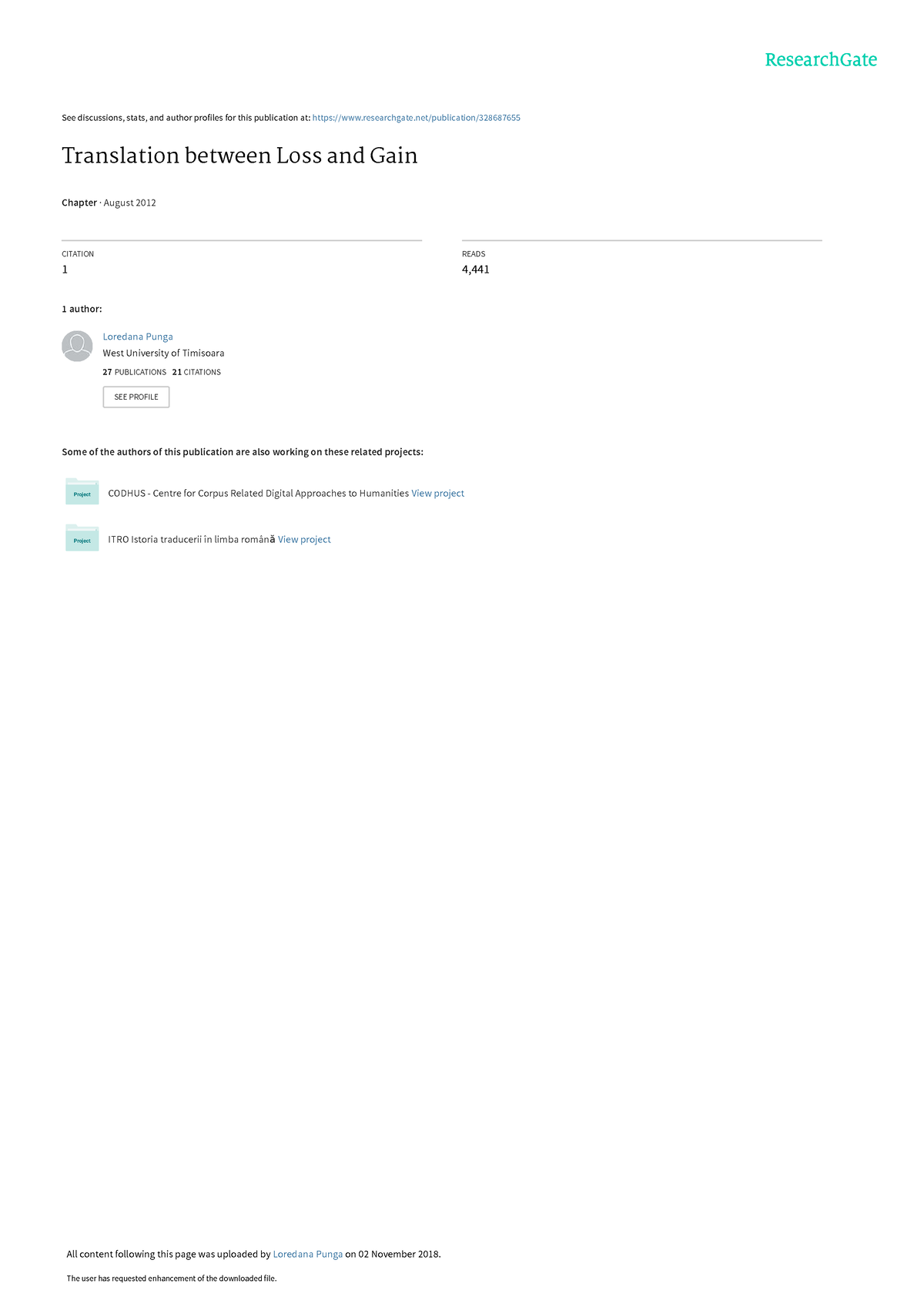This image features a stark white background with a thin horizontal line running across the top. In the upper right corner, the text "ResearchGate" is subtly printed in light blue. Below this, the phrase "A Translation Between Loss and Gain" is prominently displayed in purple. Scattered near the top are several small words and lines that are not easily readable due to their size.

On the right side, aligned vertically, is a small gray circle containing a person's profile icon and name. Directly beneath this, there is a horizontal line followed by a button for an action.

Further down, the image transitions into a sign-off section that includes two small blue squares stacked vertically, each accompanied by minuscule lines of text. The bottom portion of the image features a conspicuous blank space, with two additional diminutive lines of text positioned at the very bottom edge.